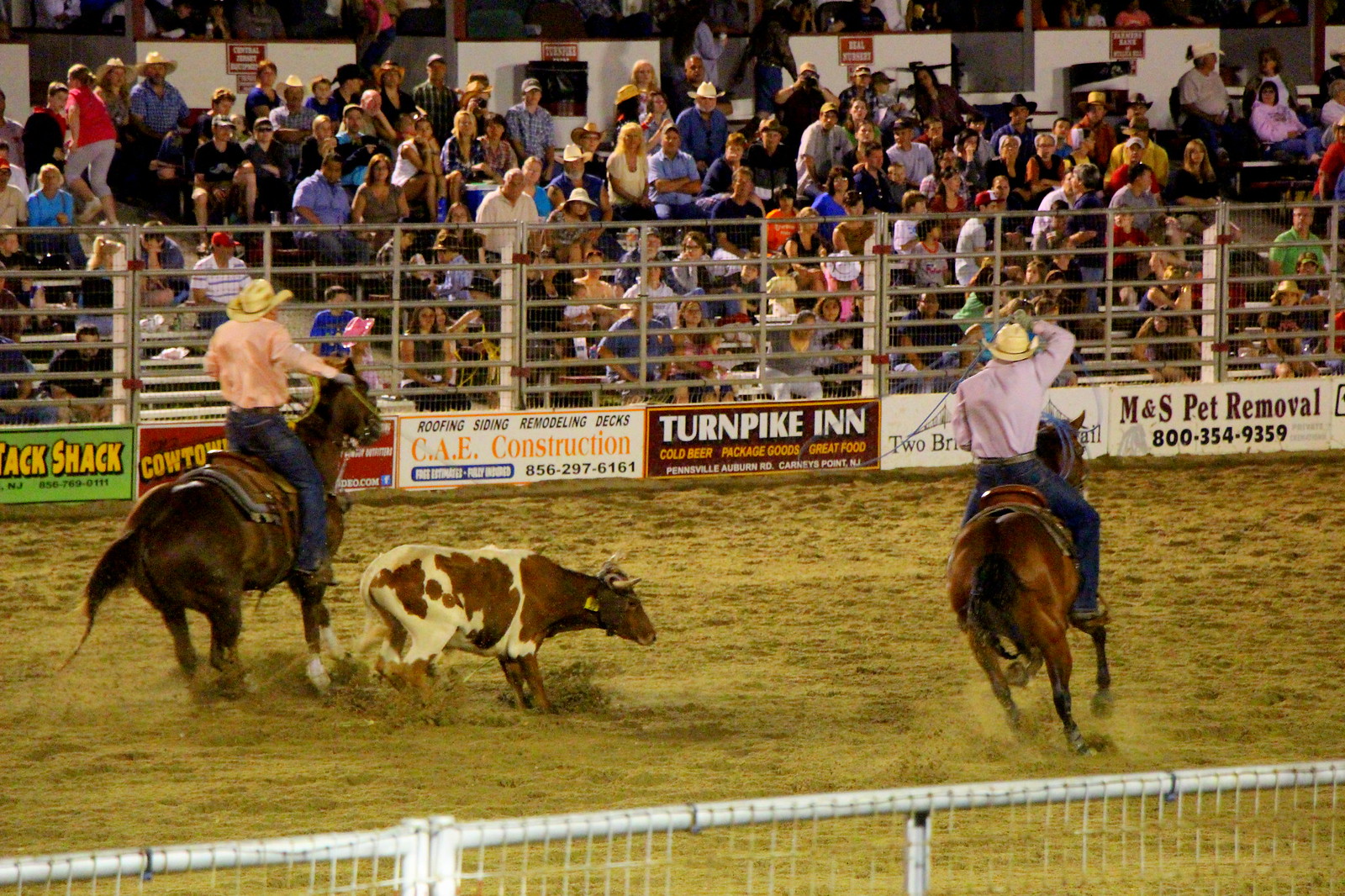The image depicts an action-packed scene from a New Jersey rodeo. In the foreground, two cowboys on horseback are engaged in a roping event. Both cowboys, wearing beige hats, long-sleeved shirts, and blue jeans, are focused on their task. The cowboy on the left, in a light-colored shirt and blue jeans, is aiming his rope at a brown and white steer, while the cowboy on the right, similarly dressed, swings his rope overhead in anticipation. Their horses are trotting on a dirt arena enclosed by a fence that runs horizontally from the bottom left and extends to the right of the image.

In the midground, another fence adorned with advertisements marks the boundary of the arena. Prominent sponsors such as Turnpike Inn, CAE Construction, Tax Shack, M&S Pet Removal, and Stack Shack are visible on the fence, indicating the event's New Jersey location. Beyond this fence, metal bleachers are packed with spectators intently watching the rodeo. The crowd and the lower deck are partially obscured by a small wall at the top of the image, emphasizing the size and scale of the event.